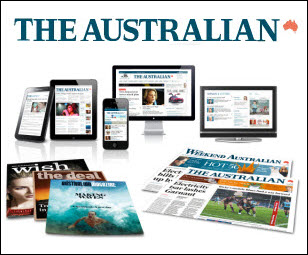A screenshot displays a predominantly white background with thin black borders, encapsulating a detailed composition. The heading "The Australian" appears prominently at the top, accompanied by a small map of Australia rendered in a reddish-orange hue. The title is written in a dark blue-green font, effectively catching the eye. 

Below the heading, a series of device images is presented: an Android tablet, a classical iPad with thick borders, an iMac, and an older iPhone, likely an iPhone 5S. To the right of these devices is a smaller Windows external display, contrasting in size to the larger iMac.

The lower section of the image features a stack of three magazines on the left. The top magazine, titled "Wish," shows a Caucasian woman with auburn hair wearing a red dress, gazing intently at the camera. Directly beneath it is a magazine called "The Deal." The third magazine, also named "The Australian," includes an indistinct subtitle to the right. 

To the right of the magazine stack are two newspapers: "Weekend Australian" and "The Australian," neatly arranged side by side.